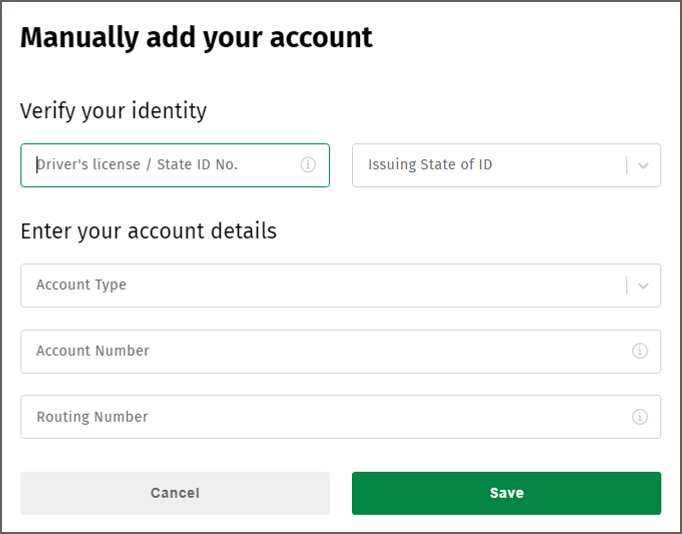The image showcases a webpage with a form for adding an account. The background of the page is white, while all text is in black. At the top left corner, a bold headline reads "Manually Add Your Account." Beneath it, in standard black text, the section prompts users to "Verify Your Identity" by entering their driver's license or state ID number, along with the issuing state of the ID, which can be selected from a dropdown menu. 

Further down, another section titled "Enter Account Details" allows the user to select the account type from a dropdown menu, and fill in spaces for the account number and routing number. 

At the bottom of the form, there are two buttons: a light gray "Cancel" button on the bottom left to abort the process, and a green "Save" button on the bottom right to submit the entered account details.

The form requires users to first provide their driver's license or state ID number, then select the issuing state, choose an account type, and finally enter the account number and routing number.